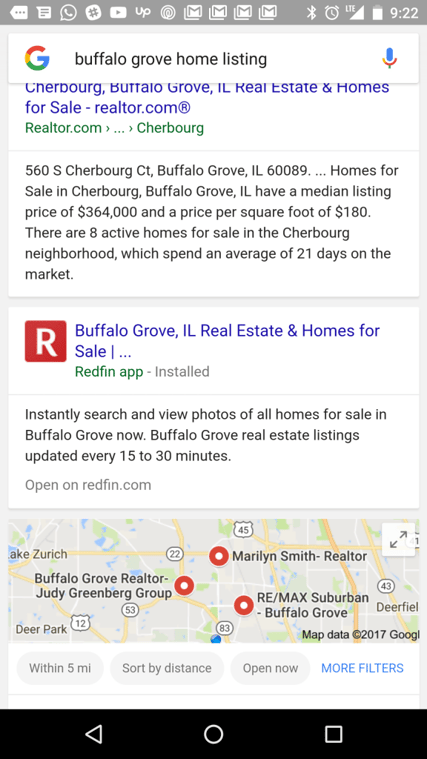**Screenshot of a Real Estate App Featuring Buffalo Grove Home Listings**

The screenshot displays a section of a real estate mobile application with several interface elements and information about home listings in Buffalo Grove, Illinois. At the top of the screen, white icons for Gmail and other common apps are visible. The header contains the Google logo, indicating that the page is integrated with Google's services, and it bears the title "Buffalo Grove Home Listings."

On the right-hand side of the header, there is a microphone icon enabling voice dictation for searches. Below the header, a series of search results appear. The first result reads "Shareboard Buffalo Grove, Illinois Real Estate and Homes for Sale Realtor.com." 

Further details about a specific listing include:
- Address: 560 South Shareboard Court, Buffalo Grove, Illinois, 60089.
- Medium listing price: $364,000.
- Price per square foot: $180.
- Active homes: 8 properties available.
- Average time on the market: 21 days.

A red square with a white "R" appears, denoting the properties listed by Realtors. Additional information mentions the Redfin app, emphasizing features such as the ability to instantly search and view photos of all homes for sale in Buffalo Grove. The app promises real estate listings are updated every 15 to 30 minutes, encouraging users to "Open on Redfin.com" for more detailed insights.

In summary, the screenshot provides a comprehensive view of home listings in Buffalo Grove, featuring key information like listing prices, market trends, and tools for home seekers to explore these properties further via the Redfin app.